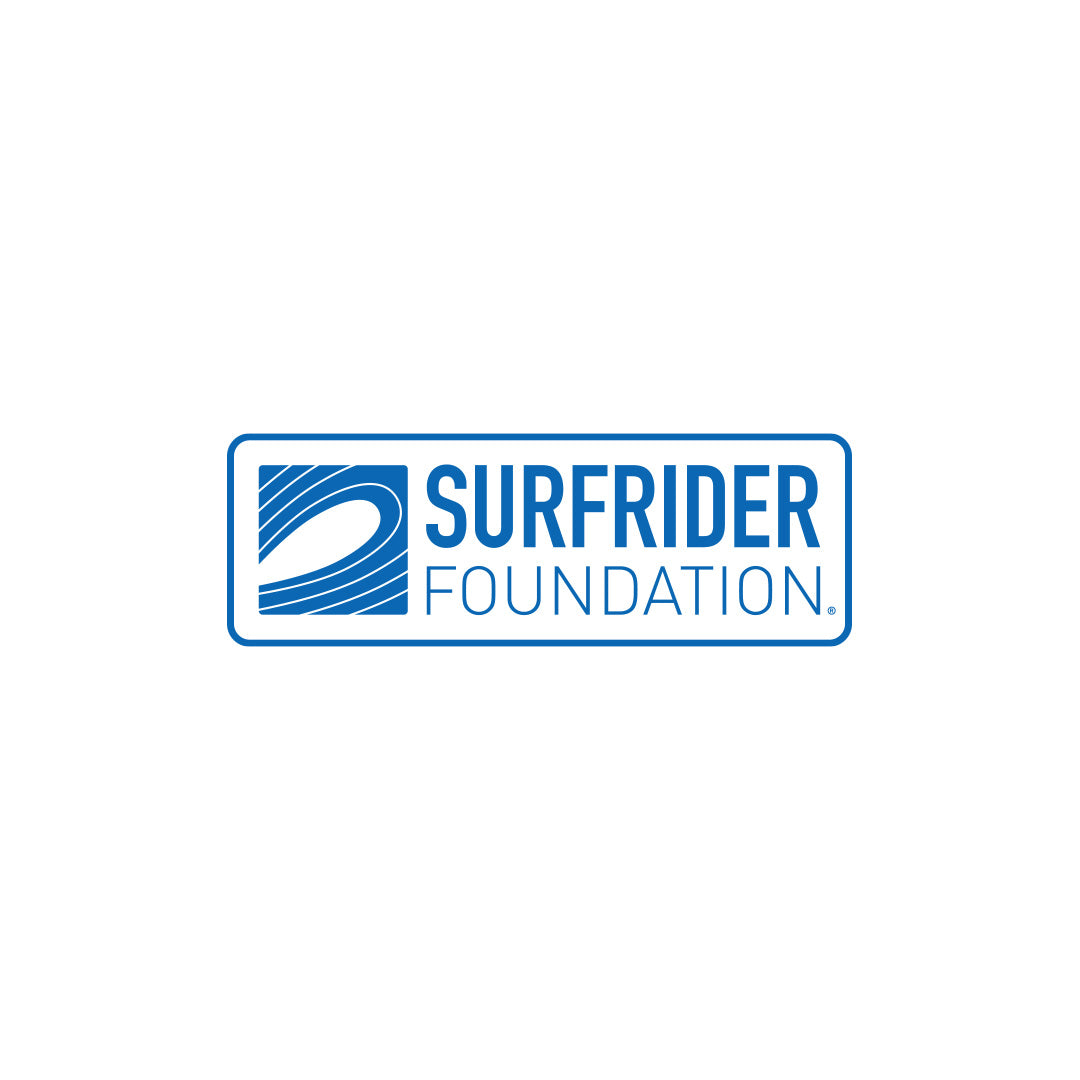The image features the Surfrider Foundation logo centered on a completely white background. The logo itself is a wide rectangle with blue borders and rounded corners. Inside the rectangle, the left side houses a square logo, which depicts blue fields with white lines that form the image of a wave, symbolizing a surfer. Next to this square, on the right, is the text "Surfrider Foundation" with "Surfrider" in large, bold blue letters, and "Foundation" beneath it in smaller, non-bold blue text. There is a copyright symbol next to the end of "Foundation." The simplicity and clarity of the design emphasize its aquatic theme and organizational identity.